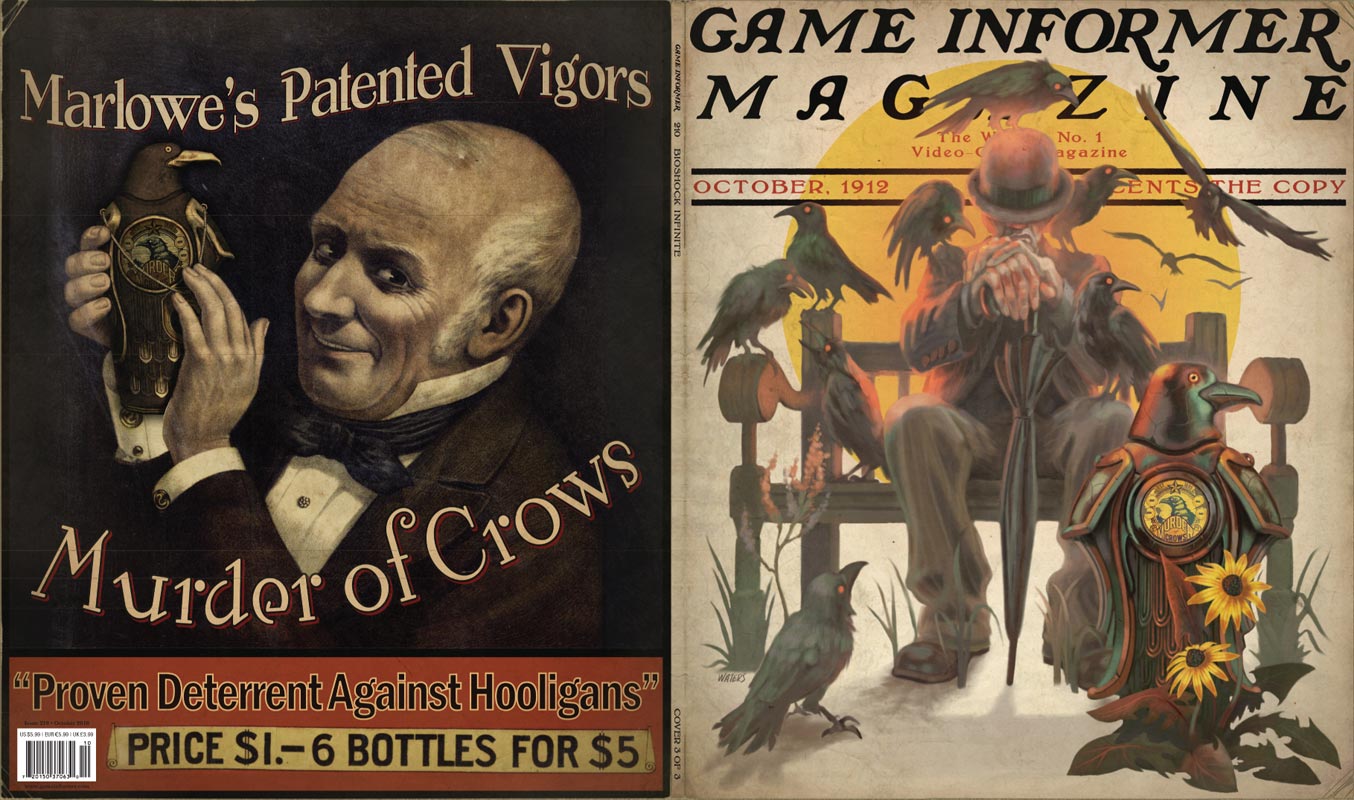The image features two distinct magazine covers side-by-side:

**Left Image**: This cover displays an advertisement styled like an early 1900s poster, with a black background and cream-colored text that reads "Marlowe's Patented Vigors." Below it, in a circular badge, it proclaims "Murder of Crows," referring to a product described as a "proven deterrent against hooligans." An older bald man with white sideburns, smiling and holding a crow-like wooden sculpture with the word "Murder" inscribed on it, dominates the image. The price is listed as "$1 for six bottles worth $5," and there's a vintage-style UPC code in the bottom left corner.

**Right Image**: This cover belongs to Game Informer Magazine and mimics the style of The Saturday Evening Post. It depicts a man sitting on a bench surrounded by crows. The man, whose face is hidden by a top hat pulled low, holds a closed umbrella upright with his hands resting on top. Crows are perched all around him: on his hat, shoulder, and even the bench. There's a large crow standing prominently in the foreground. The text includes "Game Informer Magazine" in black font and "October 1912."

Both images bear a unique retro aesthetic, blending gaming culture with vintage advertisement styles, evoking a mysterious and intriguing scene reminiscent of early 20th-century graphics.